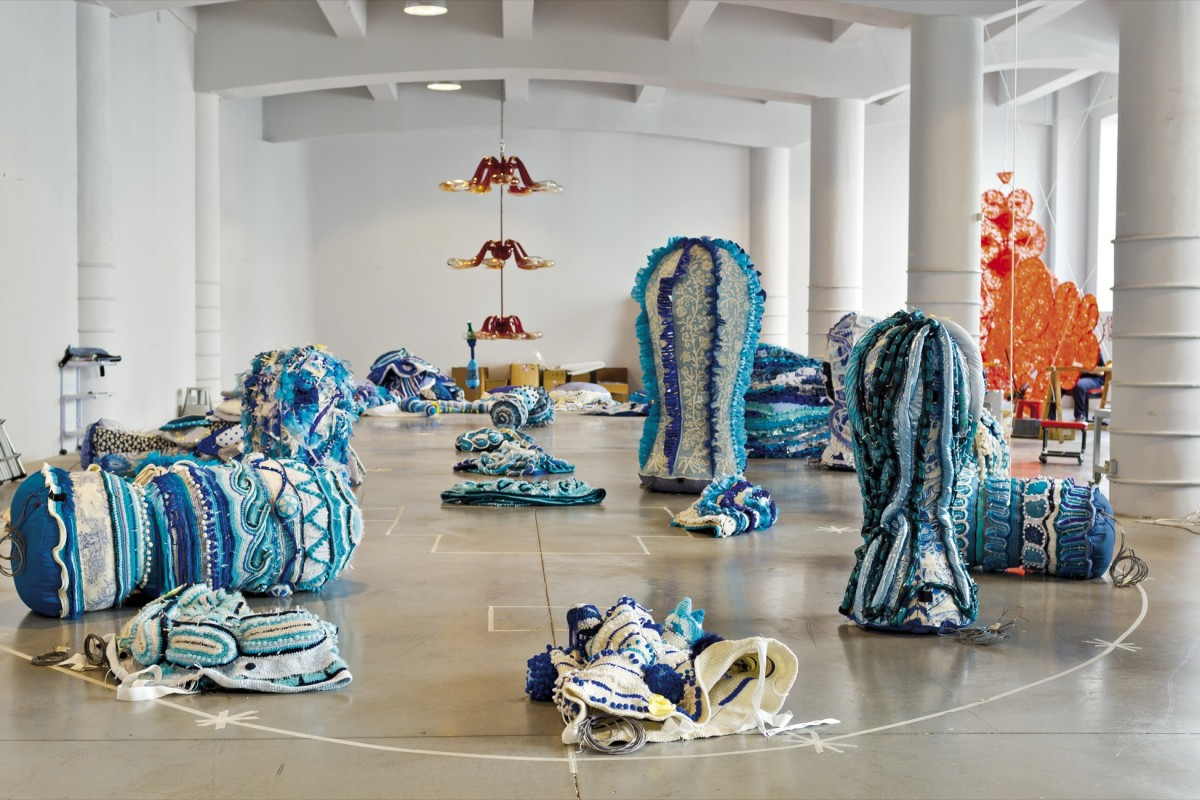The image depicts an expansive art studio with pristine white walls and several large white columns stretching down the right side of the room. The floor is a bare concrete surface. The studio is adorned with various fabric decorations, primarily in shades of blue and white, which seem to be woven together in a crocheted or knitted fashion. These fabric pieces are both piled and spread out across the space, some draped over the columns and others loosely scattered on the floor. The main artistic focus appears to be a circle of blue, bulbous structures, surrounded by tubular shapes, creating a striking visual contrast against the studio's minimalist backdrop. Additionally, there is a noticeable chandelier-like installation in the background composed of blown glass in red and yellow colors, adding a layer of vibrant complexity to the scene. Off to the right, partially obscured by the art, a person is seated near orange and red art installations, further contributing to the studio's eclectic atmosphere. The room is bathed in natural light, highlighting the intricate patterns and textures of the fabric art pieces.